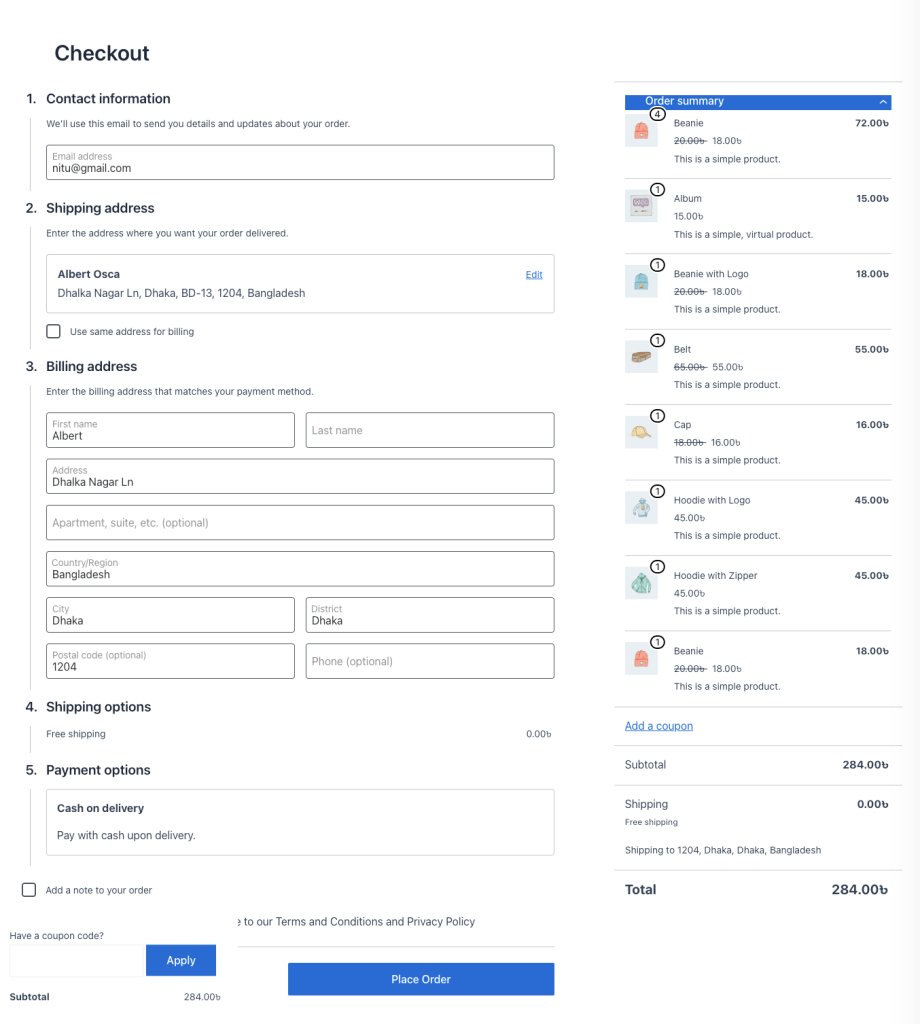### Detailed Caption of the Checkout Screen Image

The image displays a screenshot of a software checkout page, organized into five distinct sections with clear headings and subheadings.

#### Section 1: Contact Information
- **Heading:** `Checkout`
  - **Subheading:** `1. Contact Information`
  - **Text:** "We'll use this email to send you details and updates about your order."
  - **Input Box:** Labeled "Email Address" with pre-filled text `nitu@gmail.com`.

#### Section 2: Shipping Address
- **Subheading:** `2. Shipping Address`
  - **Text:** "Enter the address where you want your order delivered."
  - **Input Box:** Pre-filled with `Albert Oscar, Dhalk Nagar Ln, Dhaka, BD-13, 1204, Bangladesh`.
  - **Checkbox:** Labeled "Use same address for billing," which is unchecked.

#### Section 3: Billing Address
- **Subheading:** `3. Billing Address`
  - **Text:** "Enter the billing address that matches your payment method."
  - **Input Boxes:**
    - First Name: Pre-filled with `Albert`
    - Last Name: Empty
    - Address: Pre-filled with `Dhalk Nagar Ln`
    - Apartment, Suite, etc.: Empty (optional)
    - Country/Region: Bangladesh
    - City: Dhaka
    - District: Dhaka
    - Postal Code: Pre-filled with `1204` (optional)
    - Phone: Empty (optional)

#### Section 4: Shipping Options
- **Subheading:** `4. Shipping Options`
  - **Text:** "Free Shipping" (small text)

#### Section 5: Payment Options
- **Subheading:** `5. Payment Options`
  - **Text:** "Cash on Delivery"
  - **Description:** "Pay with cash upon delivery."
  - **Checkbox:** Labeled "Add a note to your order," followed by the text "Have a coupon code?"
  - **Button:** Large blue "Apply" button
  - **Disclaimer:** "Terms and Conditions and Privacy Policy" (fine text)
  - **Button:** Large blue "Place Your Order" button

#### Order Summary
- **Section Heading:** Blue header labeled "Order Summary"
  - **Items Listed:** Each divided by a thin line with item name, price, and icon.
    - **Beanie:** 72.00B
    - **Album:** 15.00B (with description "A simple virtual product")
    - **Beanie with Logo:** 18.00B
    - **Belt:** 55.00B
    - **Cap:** 16.00B
    - **Hoodie with Logo:** 45.00B
    - **Hoodie with Zipper:** 45.00B
    - **Beanie:** 18.00B
  - **Subtotal:** 284.00B
  - **Shipping:** Free shipping (0.00B) to `1204 Dhaka, Dhaka, Bangladesh`.
  - **Total:** 284.00B

Each part of the form is meticulously organized, providing clear instructions and pre-filled example data to illustrate the intended input. The overall layout is user-friendly, with essential call-to-actions like "Apply" and "Place Your Order" prominently highlighted.